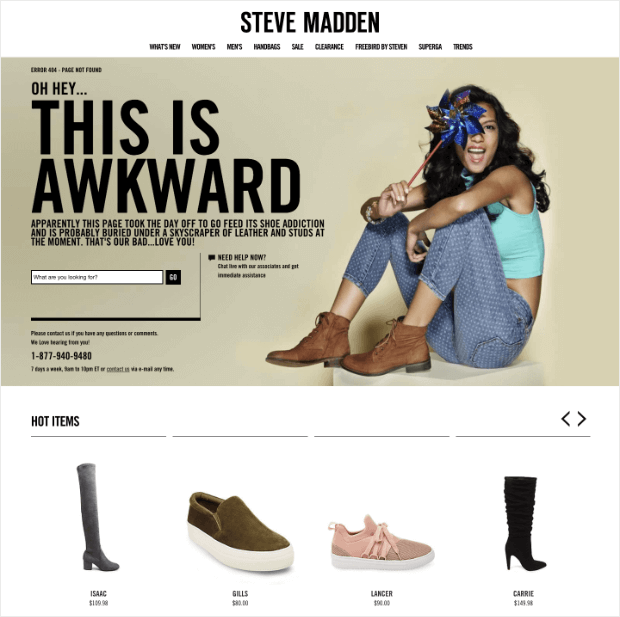A screenshot from the Steve Madden website showcases the brand's logo prominently at the top in bold, black, all-caps text. Below the logo, nine menu options are centered and displayed in smaller bold, black text, though too small to read clearly. The main content area features a beige rectangle with an eye-catching introduction in bold, black, all-caps text reading "OH HEY..." followed by "THIS IS AWKWARD" in larger bold, black text on the next line. Underneath, three lines of smaller black text are visible, though the content is not specified.

Approximately four rows down, a search bar is positioned, and to its right is an image of a woman. She has long dark hair and is holding a small blue pinwheel. The woman is seated with her knees drawn up to her chest, her arms resting on her knees. She is dressed in brown boots, blue jeans, and a cropped light green top.

Directly below the beige rectangle on the left, bold, black text reads "HOT ITEMS," accompanied by left and right pointing arrows on the right side. Beneath this section are four light gray horizontal lines. Featured below the lines are images of footwear: from left to right, a boot, a flat brown shoe, a pink sneaker, and a black high-heeled boot.